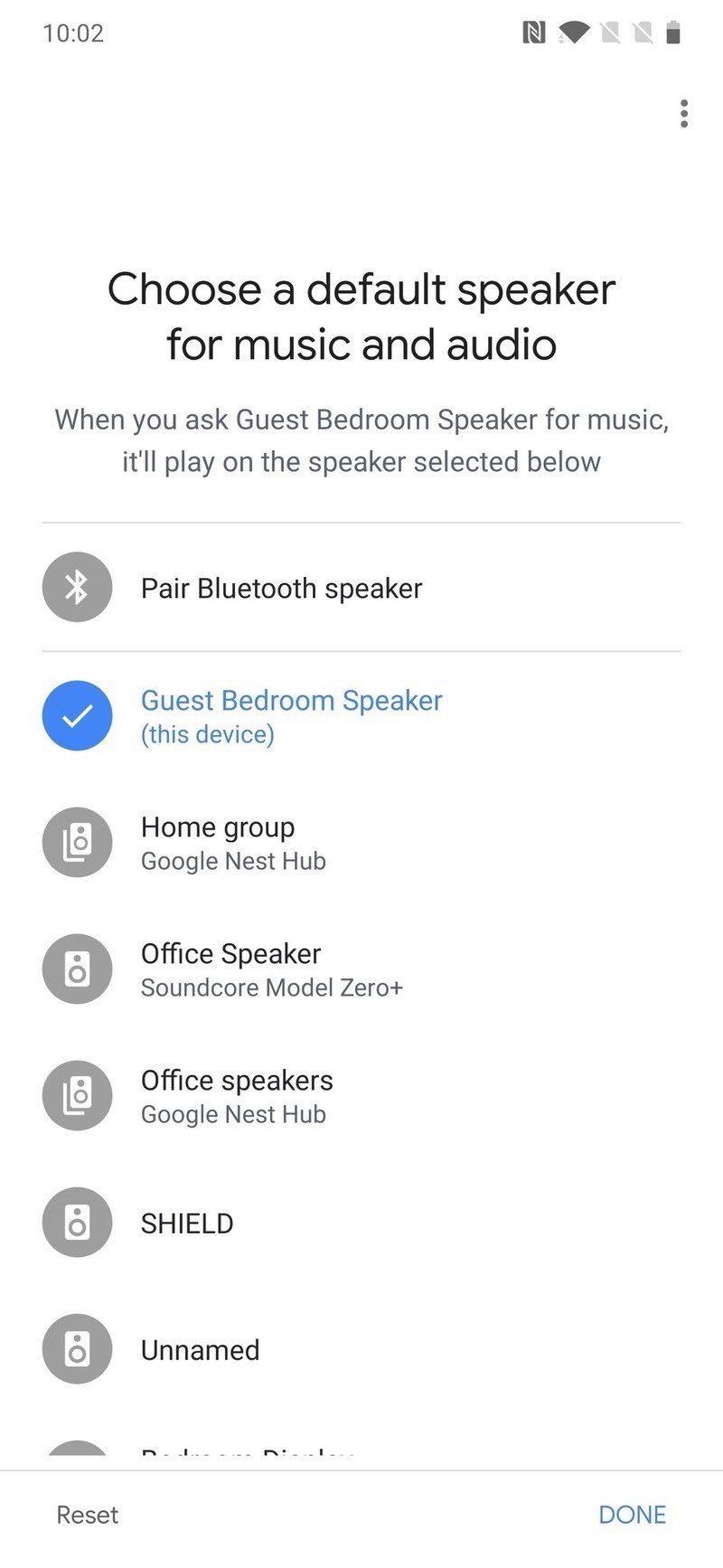The image is a screenshot of the "Like Settings" section within an app. The screenshot was taken at 10:02, as indicated by the time displayed at the top left. On the right side of the top bar, the status icons are visible, including the Wi-Fi icon, two grayed-out battery icons, and a regular battery icon.

In the main content of the screen, the title at the top reads, "Choose a default speaker for music and audio." Below this title, there is a description that states, "When you ask Guest Bedroom Speaker for music, it'll play on the speaker selected below."

Following the description, there is an option to "Pair Bluetooth Speaker." Under this option, a list of available devices is displayed:

1. Guest Bedroom Speaker (highlighted with a blue color)
2. This device
3. Home group
4. Google Nest Hub
5. Office Speaker
6. Soundcore Model Zero Plus
7. Office Speakers
8. Google Nest Hub
9. Shield
10. Unnamed (the last one is partially cut off)

The detailed layout and information clearly outline the configuration options for selecting a default speaker within the app.